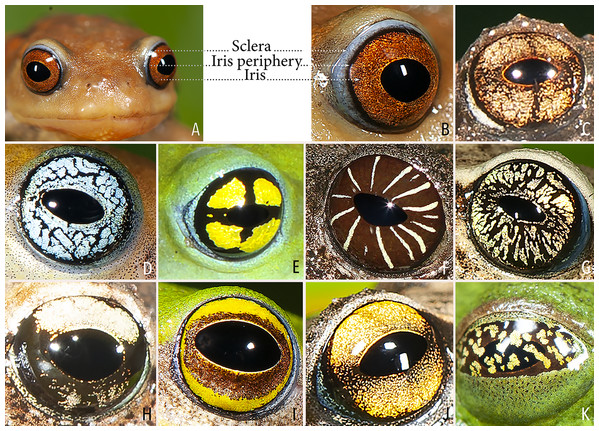This image is a detailed collage highlighting various close-up shots of frog eyes. In the top-left corner, there is a full image of a tan frog with reddish eyes and large black pupils. Adjacent to this, there are three dotted lines leading to the first of many eye close-ups, each labeled with “sclera,” “iris periphery,” and “iris.” The image contains a total of 11 close-up shots of eyes arranged in rows, labeled A to K. The eyes display a wide range of colors and patterns – from green and yellow to black, brown, blue, and more. Some eyes have distinct patterns resembling a glazed chocolate donut with white lines, others showcase splattered lines or clustered blobs. The background of the image is white, enhancing the vivid eye colors and intricate details.